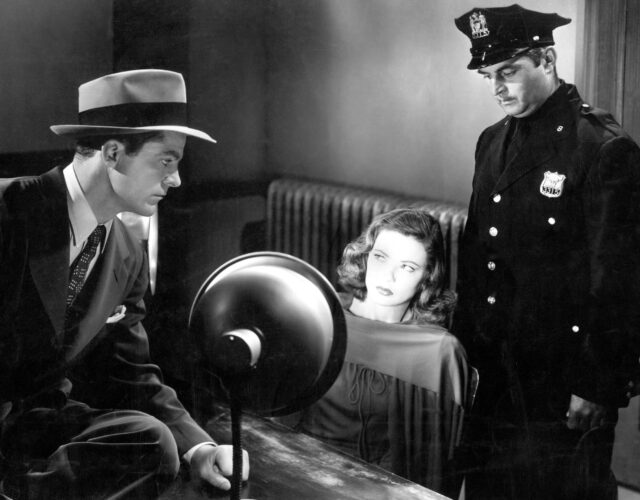In this atmospheric black-and-white photograph, set in a small, dimly lit room that evokes the 1950s or 60s, three figures create a tense tableau. A detective, clad in a dark suit, tie, collared shirt, and wearing a fedora, leans with one knee on a wooden desk, staring intently at the woman seated before him. The harsh beam of a desk lamp casts an unforgiving light on her apprehensive face, revealing the curls at the end of her long hair. She wears a dress and sits in a plain metal chair, looking up anxiously at the detective, clearly the focus of an intense interrogation. To her right and slightly behind, a policeman in full uniform, complete with hat and badge, stands watchfully. The room itself is sparse, with a radiator along one lighter-colored wall, contrasting with the dark trim, a door positioned behind the policeman, and a small desk and cabinet adding to the spartan setting. The scene, likely a still from a film or TV show, captures a moment fraught with tension and drama.